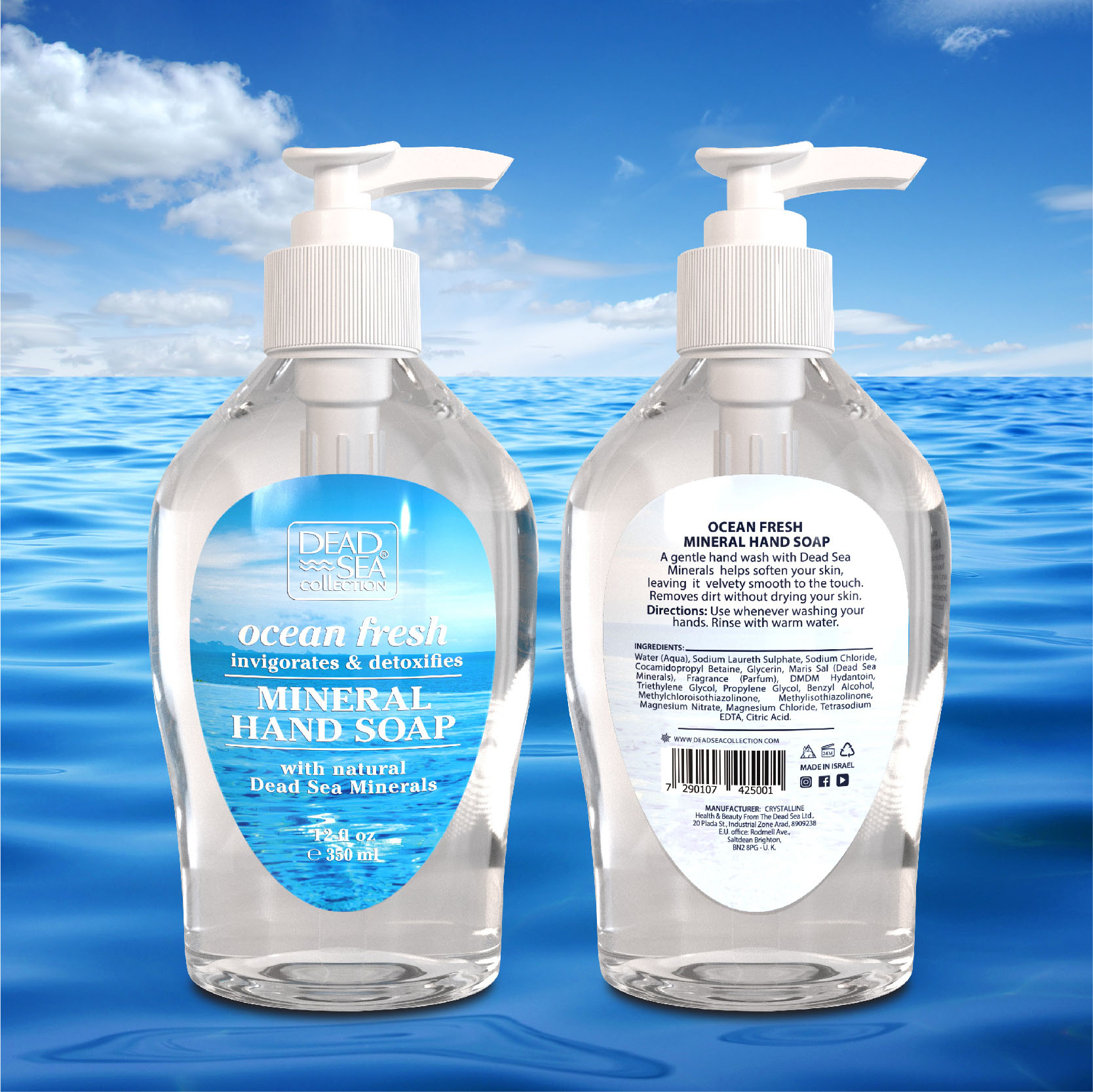An advertisement for Dead Sea Collection's Ocean Fresh Mineral Hand Soap is depicted, featuring both the front and back views of the product bottles against a digitally manipulated backdrop of an endless blue ocean and a sky dotted with patchy clouds. The hand soap's label displays a matching ocean scene, with the text "Dead Sea Collection" and "Ocean Fresh Invigorates and Detoxifies" prominently showcased. The front label describes it as "Mineral Hand Soap with Natural Dead Sea Minerals" and specifies the volume as "12 fluid ounces (350 milliliters)." The back label details that this gentle hand wash, enriched with Dead Sea Minerals, helps soften skin, leaving it velvety smooth, and effectively removes dirt without causing dryness. Additional label information includes blurry ingredients, a website, a barcode, a likely "Made in Israel" sticker, and illegible manufacturer details.